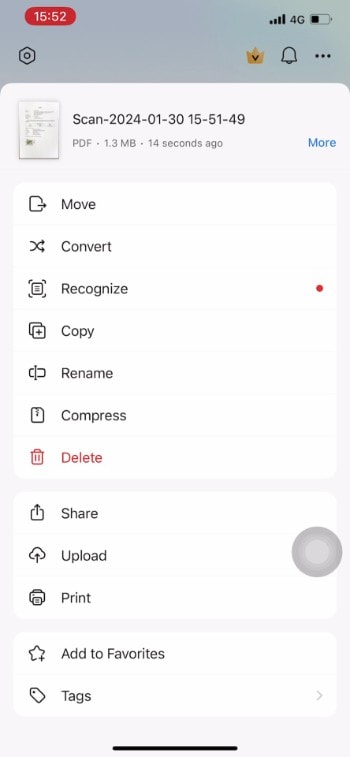This image captures a screenshot from an Android device. At the top left corner, there is a red oval displaying the number 1552. On the top right, various status icons are aligned in a row, including the Wi-Fi signal, a 4G indicator, and a battery icon showing a 50% charge. Below these, on the left, is a settings cog, and to its right, a crown icon with a down arrow. Following this, a bell icon and three vertical dots appear sequentially.

The main section of the screen shows detailed information, starting with a timestamp labeled "scan 2024-04-30 15-51-49." To the left of this text is a thumbnail preview of the scanned image. Beneath the scan details, it states "PDF 1.3 MB" with a time indication of "14 seconds." There is also a blue highlighted option labeled "more" on the right.

At the bottom of the screen, a row of actionable icons is divided into three sections. The first section includes options to "move," "convert," and "recognize." The second section starts with "share," followed by two more items not fully visible. The final section contains "add to favorites" and "tags."